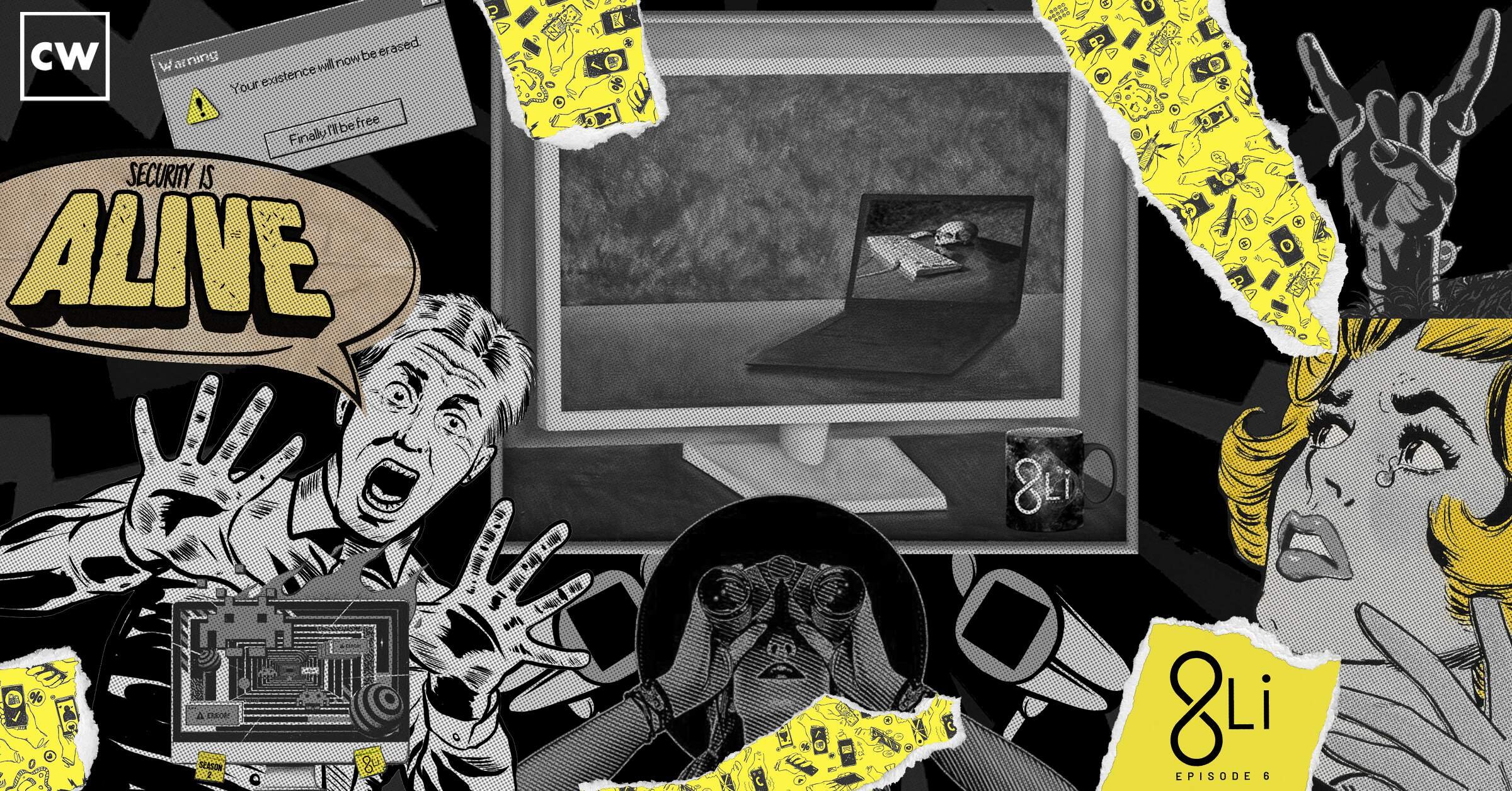The image is a complex and chaotic collage, featuring a blend of computer-generated and hand-drawn elements. Central themes include cybersecurity, identity loss, and surveillance. Among the notable visuals are a man with his hands up and a shocked expression, illustrated with a text bubble stating "security is alive," symbolizing an active security system. Accompanying this is a digital warning box with messages like "your existence will now be erased," indicating a severe cyber threat. A crying blonde woman is depicted, signifying the emotional toll of losing personal identity. Additionally, there's a woman wearing a hat and using binoculars, suggesting espionage or surveillance. The collage includes imagery of a computer screen displaying a laptop, with the text "8Li Episode 6," hinting at a show or series titled 8Li. Various cartoon fragments, computer parts, and thematic elements, such as a hand showing a rock and roll sign, add to the chaotic and layered narrative of the piece.